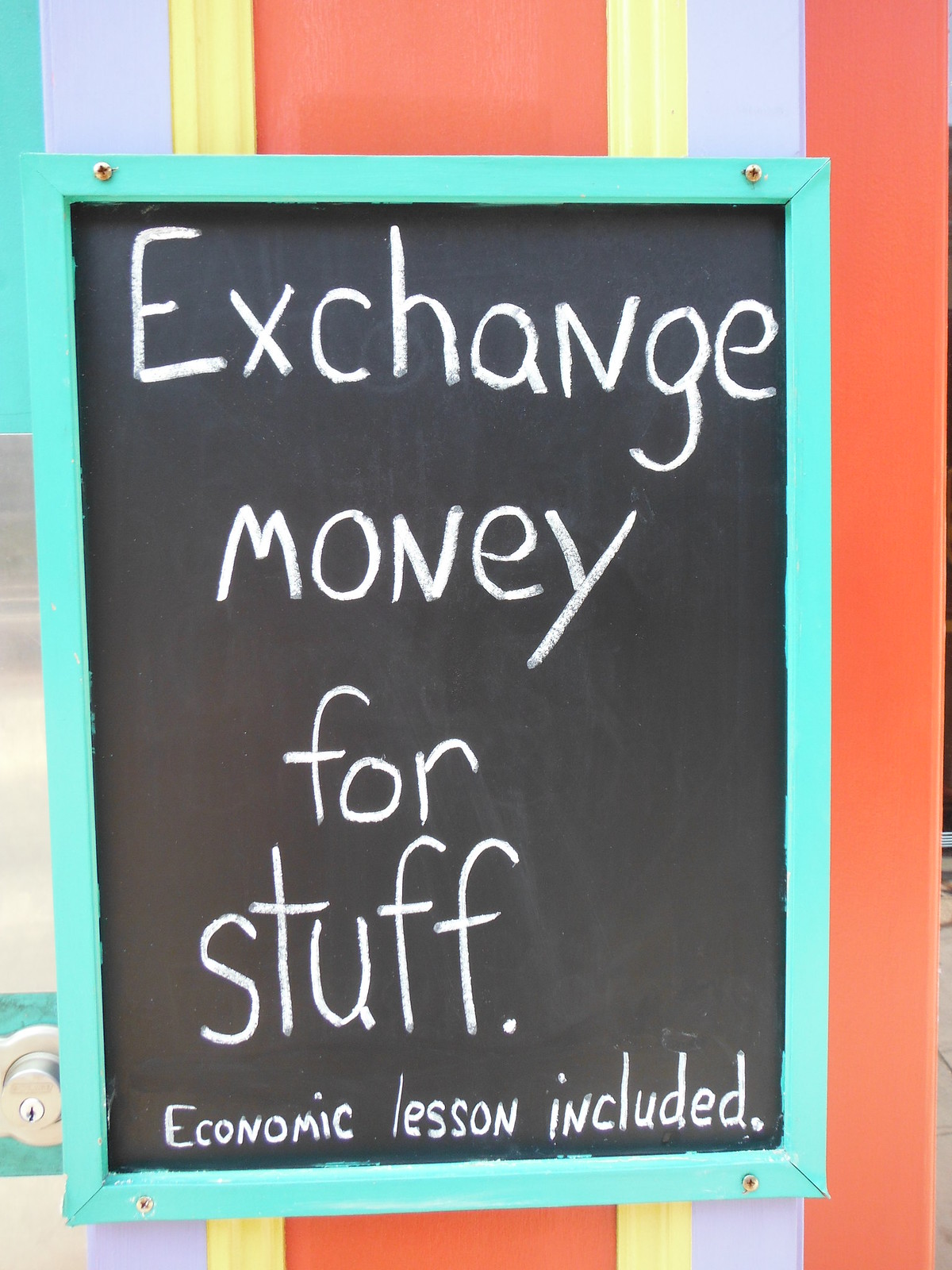The image showcases a handmade rectangular blackboard with a bold sky blue border secured by screws in all four corners. In white chalk handwriting, the board reads, "Exchange money for stuff" and "Economic lesson included." The handwriting appears informal and childlike. The blackboard is mounted on a wall featuring an eclectic mix of colors, including vertical stripes of light lavender, peach, and yellow. Additionally, an orange panel is visible on the right, and a silver doorknob partially crops out on the left side, suggesting a door nearby.